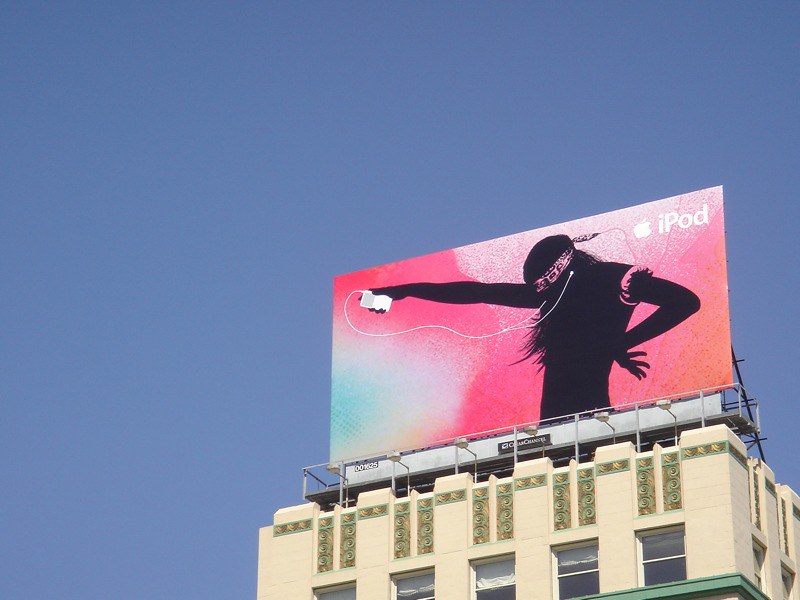This photograph, taken from street level during the daytime, captures a multi-story, cream-colored apartment building with a clear blue sky as the backdrop. The building is viewed slightly from the right, showing five front-facing windows and two windows curving down the right-hand side. At the top, the building features five decorative brickwork motifs, and a green ledge runs beneath the fourth and fifth windows. Dominating the scene is a large billboard atop the building, mounted on scaffolding. The billboard features a vibrant, mostly pink watercolor-style background with splashes of orange, blue, and white. The focal point is a silhouette of a woman with long hair and a pink bandana, extending her right arm to hold a white iPod, its wire trailing to her ears. Her left arm is bent, with her hand near her back. In the upper right corner of the billboard, the familiar Apple logo and the word 'iPod' are prominently displayed in white. A small black rectangle at the base of the billboard says "Clear Channel." Overall, the image combines urban architecture with iconic advertising against a cloudless sky.